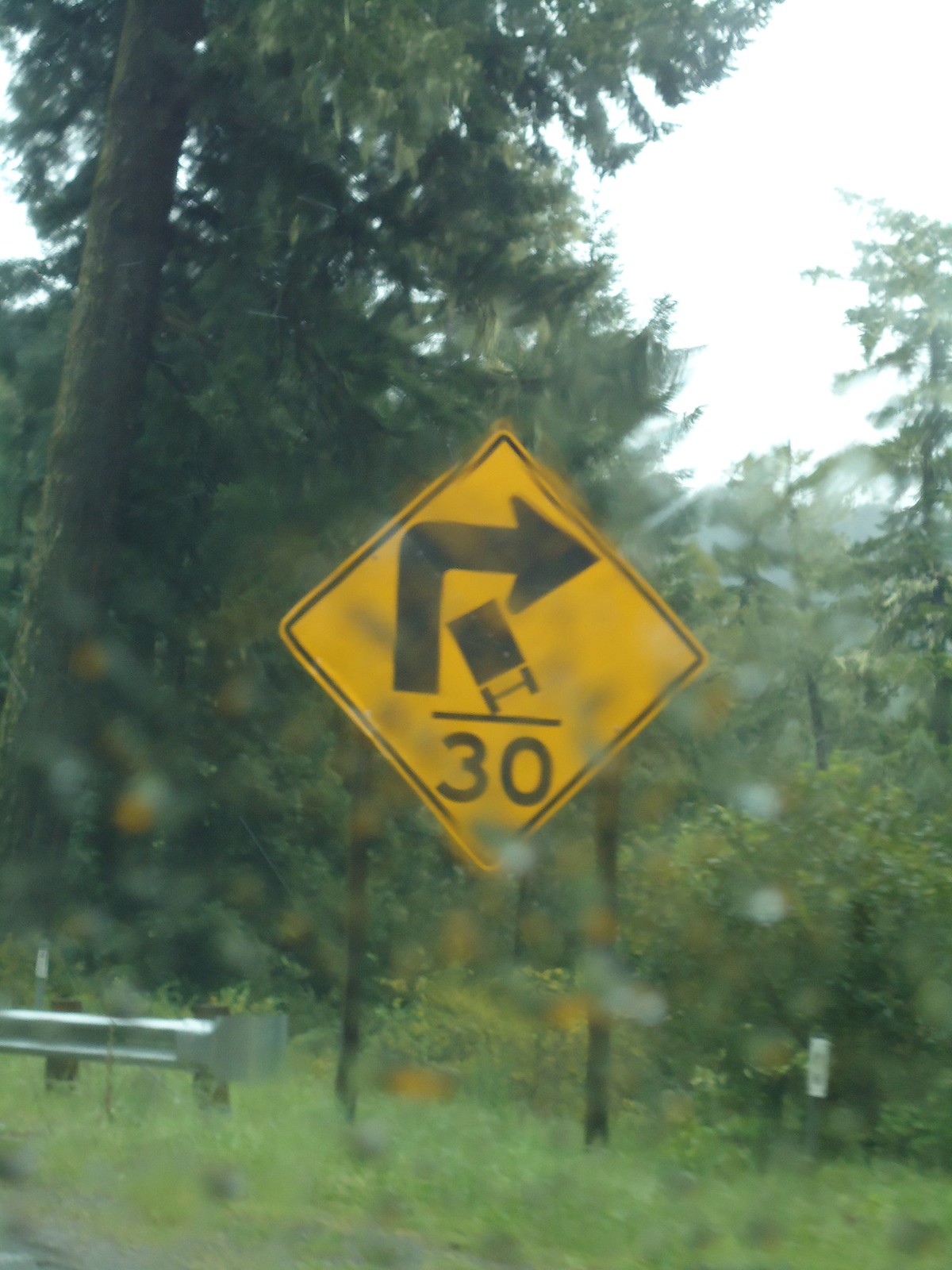This outdoor photograph, likely taken from inside a vehicle on a rainy day, captures an evocative scene through a rain-speckled window. Central to the image is a yellow diamond-shaped highway sign, featuring a black arrow that ascends before sharply turning to the right, accompanied by the number "30." The backdrop reveals a lush forest of tall, verdant trees, indicative of spring or summer. The ground is carpeted with vibrant green grass, contributing to the overall freshness of the scene. In the image's bottom left corner, a shiny silver metal road barrier is visible, adding to the sense of location and roadway safety. The rain-blurred view enhances the mood of the day, emphasizing a serene yet slightly melancholic ambiance.